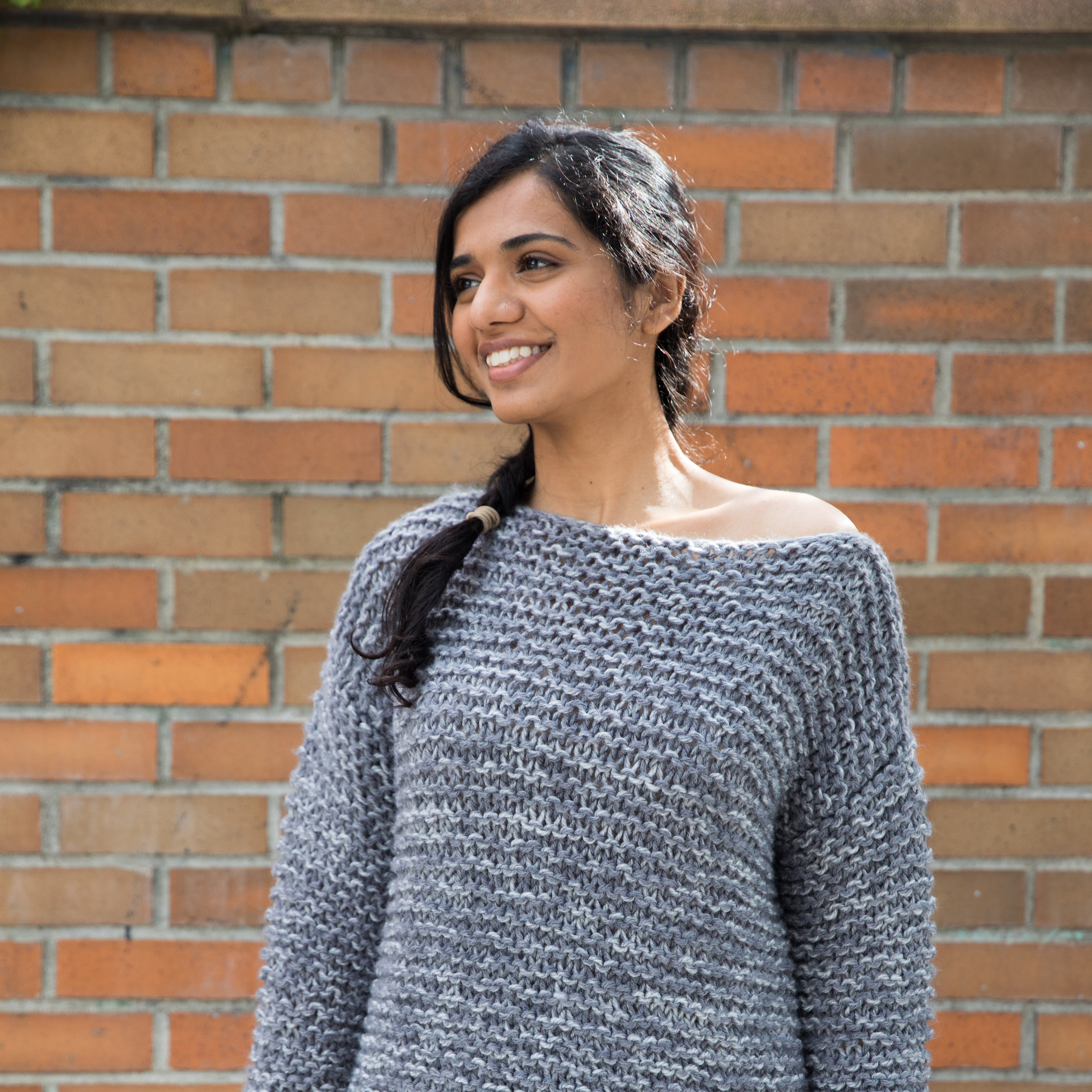In this close-up quality photograph, a young woman, appearing to be in her early 20s, stands in front of a brick wall with a mix of brown and orange hues. She has darker, olive-toned skin, possibly of South Asian or Hispanic origin, and sports a bright smile as she gazes off to her right. Her dark black hair is styled in a braid that cascades over her right shoulder, secured with a tan rubber band, and the braid ends in soft curls. She also has bangs that frame her face. Her eyes are round and almond-shaped, complementing her distinct Eastern Asian Indian features. She wears a gray, chunky knitted sweater with a thick braided texture, made possibly of yarn or tweed. The sweater covers her right shoulder and arms but hangs off her left shoulder, revealing her collarbone and part of her shoulder. The sunlight appears to illuminate the left side of her body, enhancing the warmth of her smile and the rich details of her attire.